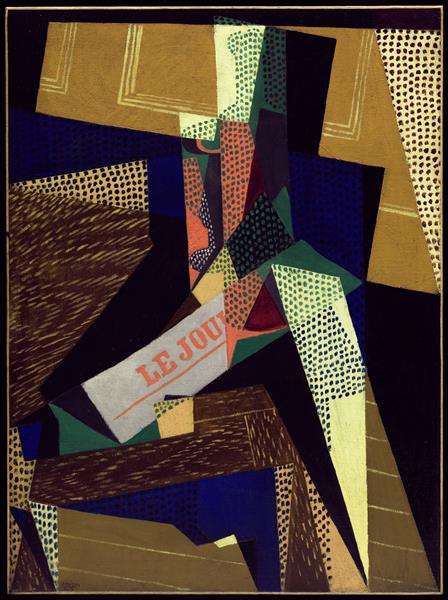This image appears to be a highly abstract, cubist-style painting, characterized by a complex assembly of overlapping shapes and patterns against a black background. Dominated by an arrangement of rectangles, the artwork features a range of colors including brown, tan, dark blue, light yellow, green, and red, with several shapes textured to resemble wood and others peppered with black dots. At the focal point of the composition, a gray rectangle bears the partially visible text "LEJOU," suggesting a possible reference to a newspaper, though the word is cropped and incomplete. The entire image is layered in such a way that elements appear to overlap and create a three-dimensional effect, with the various shapes and patterns seemingly floating at different angles. The painting is further framed by a thin tan line which subtly contains the dynamic, abstract composition. Overall, it embodies a profound sense of artistic abstraction and intricate design.